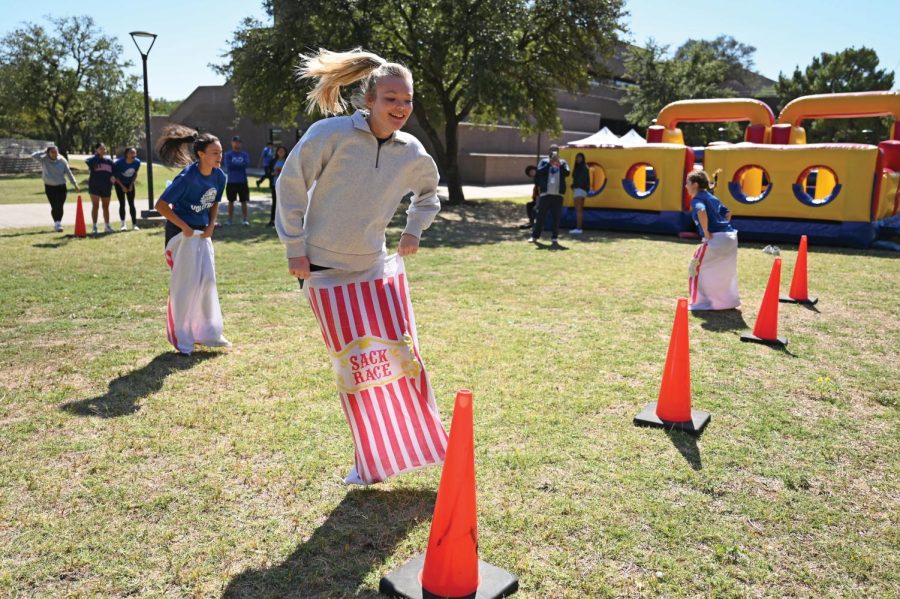In the image, a lively scene at a school fair features a classic sack race taking place on a grassy field. Three young girls, their hair tied up in ponytails, compete in the race, each jumping energetically in white sacks adorned with red pinstripes and the words "sack race" in red lettering. The girl closest to the camera, wearing a gray sweatshirt and sporting long blonde hair, smiles brightly as she hops forward. Another girl with long black hair and a blue shirt follows behind, while a third girl with long brown hair and a blue shirt appears to pull ahead, having already turned towards the finish line. The race progresses towards four orange cones lined up on the right side of the frame. In the background, a colorful inflatable playground with yellow, red, and blue hues creates a festive atmosphere, while several spectators, including someone capturing the moment with a camera, cheer the competitors on. The scene is dotted with green trees, a lamppost, and a dark brown building that is likely the school. The clear blue sky overhead completes the vibrant setting.